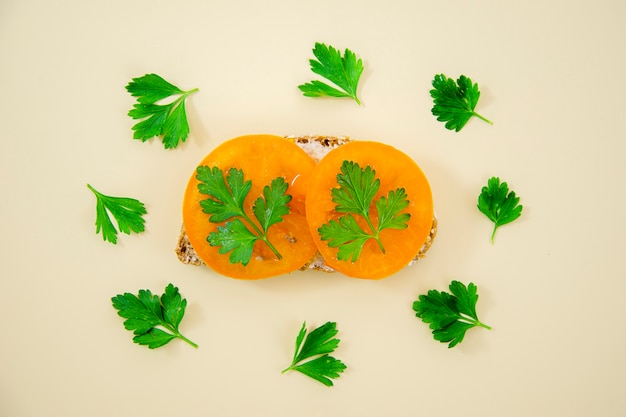This overhead image features a beautifully presented piece of toast, lightly coated with what appears to be cream cheese, though only small portions of the spread are visible. Resting on the toast are two circular slices of tomato, which are a light orange color indicating they might not be fully ripe. Each tomato slice is topped with fresh, vibrant green parsley leaves, arranged with their stems pointing towards the top left. Surrounding the toast are eight additional parsley leaves, spaced evenly in an oval semi-circle pattern, creating an aesthetically pleasing arrangement. The entire composition rests atop a tan, off-white surface, adding to the natural and fresh presentation of the dish.